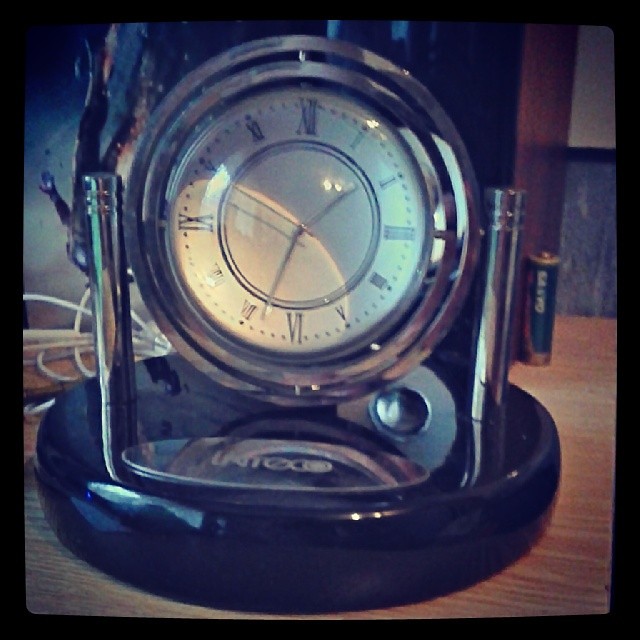A vintage-inspired table clock with a glossy black cylindrical base and a lustrous chrome metal body stands elegantly on a wooden table. Its round, pristine white face features Roman numerals marking the hours, while the classic black hour and minute hands point towards 1:50, indicating it is ten minutes to two. The clock’s sophisticated design and gleaming finish add a touch of timeless charm to its refined setting.